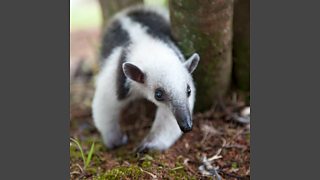The image showcases a small, possibly elusive mammal resembling a badger or anteater. It is a close-up photograph capturing the animal's distinct features and its natural environment. The creature is facing towards the camera but gazing slightly to the right. Its head is elongated and flat, with a prominent black nose at the tip of a long gray snout. The animal's eyes are black, and its ears, which stick up, are gray. The head is predominantly white, with a gradient that transitions to dark colors toward the nose.

The mammal’s body is marked by white fur interspersed with gray shades. It has white legs with two notable gray stripes on its shoulders. Its hind legs are gray with a distinct white stripe running down its back, adding to its unique pattern. The photograph captures the animal as it walks through a forest floor, composed of dirt and patches of grass. A small tree trunk or plant stalk appears in the background, partially framed by the animal. The scene suggests a natural habitat, but there is a slight indication that it might be a controlled environment such as an enclosure. The overall image is framed with a gray border, highlighting the detailed and serene moment of this creature in its habitat.